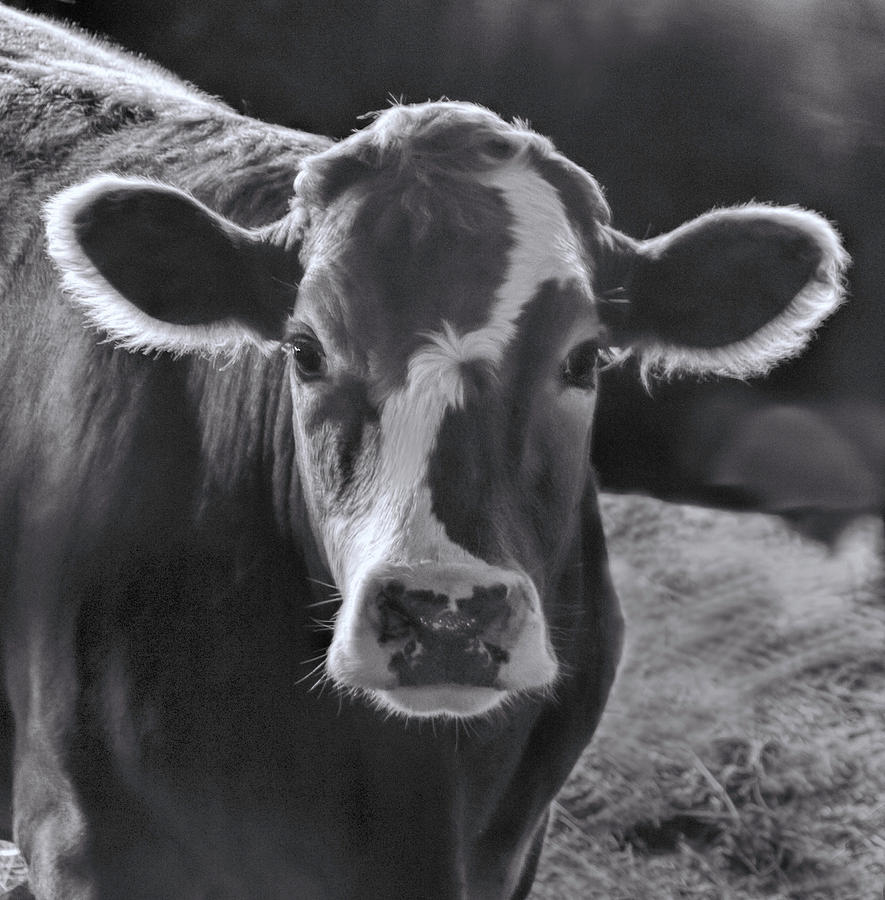This black-and-white vertical-rectangular image features a close-up of a cow's face, with only the front half of its body visible against a dark, blurred background. The cow's calm eyes are staring directly into the camera. A striking diagonal white streak runs from the left side of its forehead down across its large, dark nose, encircling it to form a distinctive white circle around the nose and mouth area. The cow's ears appear to have a white fringe, possibly due to backlighting. Scattered hay on the right side of the image suggests the cow is inside a barn. The rest of the cow's fur appears to be a uniform color, likely brown, though the black-and-white nature of the photo makes it hard to determine precisely.